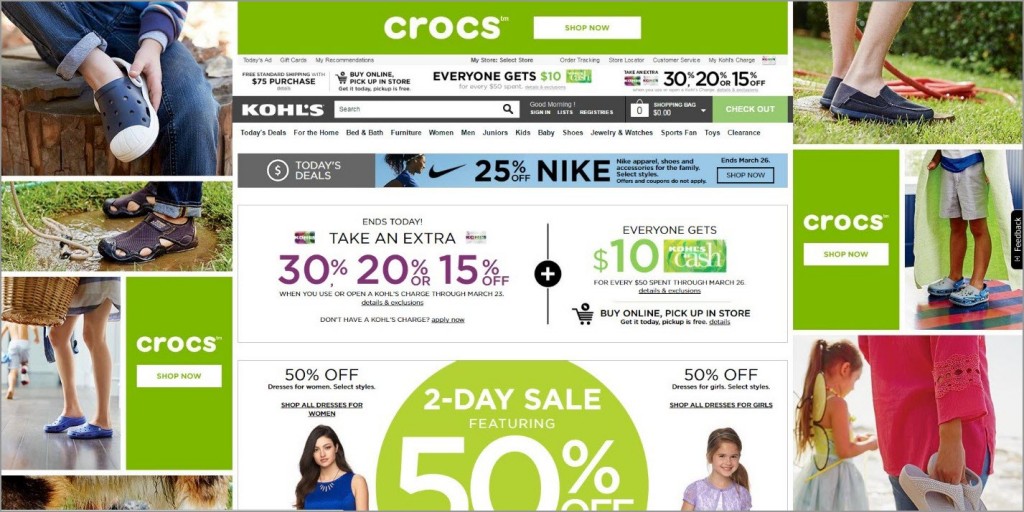Here is a cleaned-up and detailed caption for the image:

---

This promotional image from Kohl's prominently features the Kohl's logo next to the search bar at the top center of the page. The headline "Crocs" is displayed along with the specific model "Avra Tyson Crocs" and a "Shop Now" call-to-action in a white box. The top of the image captures a woman trying on a pair of blue Crocs. Additionally, there is an inset image on the left side showing someone standing in a mud puddle while wearing Crocs.

Midway through the image, a promotional banner advertises a special offer: "Everyone gets $10 off," alongside discounts of 30%, 20%, and 15%. To the right, there's another image featuring shoes, possibly Crocs, near someone holding a garden hose. Below this, a child in a bathing suit with a towel around them stands next to someone in a red shirt. This person, likely holding Crocs, is on a beach, wearing jeans and standing next to a little girl in a blue dress with wings on her back. 

At the bottom of the image, there is a prominent advertisement for a two-day sale offering 50% off, accompanied by additional offers: "Take an extra 30%, 20%, or 15% off" and "Everyone gets $10 back in Kohl's Cash." There's also a section highlighted in blue at the center that mentions "Nike" and shows a 25% discount under Kohl’s deals for the day.

---